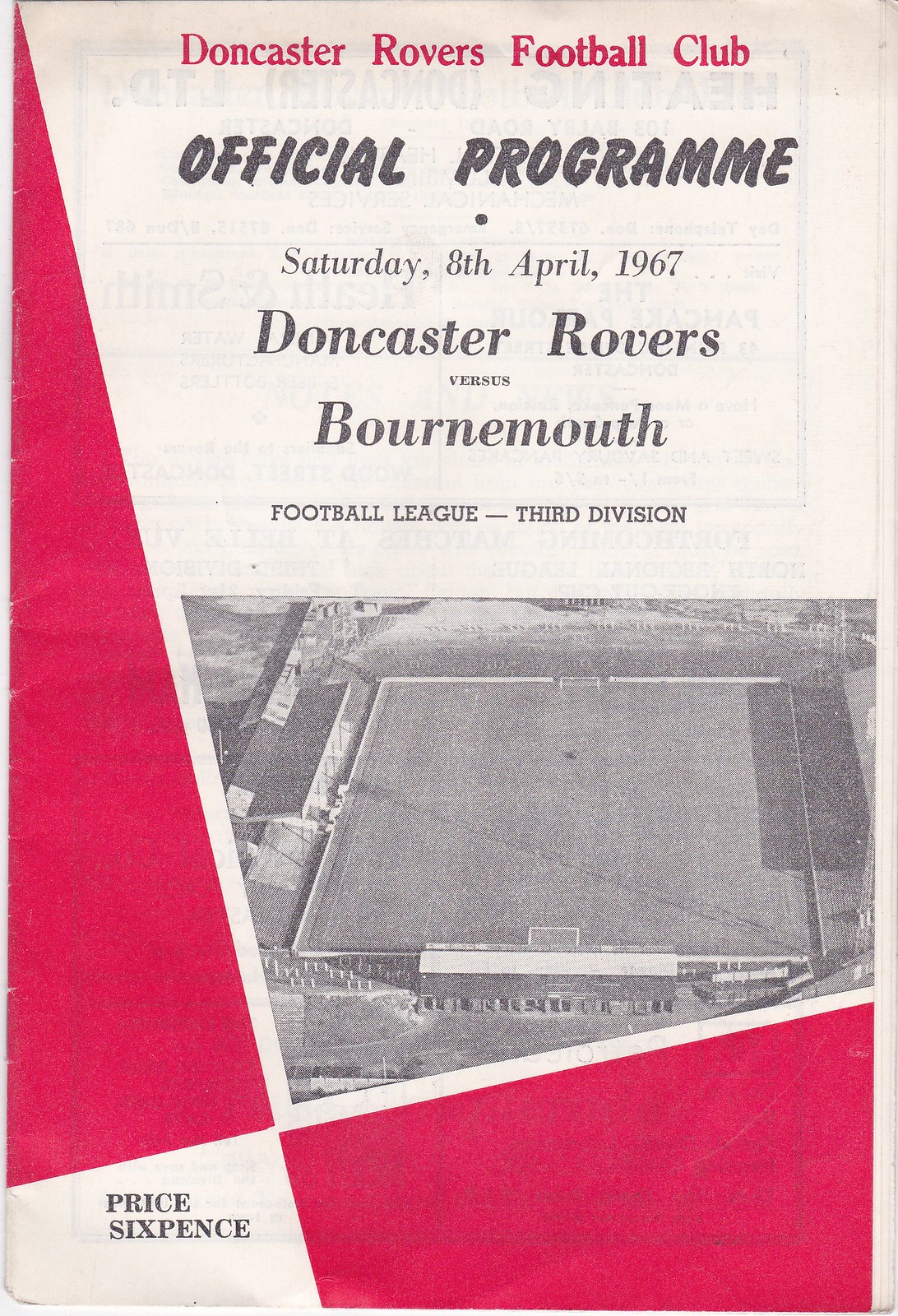The image is an old-timey cover of an official program from the Doncaster Rovers Football Club, dated Saturday, April 8, 1967. It is primarily a white cover featuring red triangular geometric designs along the left-hand side and the bottom right, creating a checkerboard effect, with the bottom left corner remaining white. At the top, it reads in red text, "Doncaster Rovers Football Club," with the remainder of the text in black: "Official Program, Saturday, 8th April, 1967, Doncaster Rovers vs. Bournemouth, Football League, 3rd Division." In the bottom left corner, it states the price as "Sixpence." A bird's eye view of a soccer field and the stands, captured from an aerial perspective, is prominently displayed in the center. The overall layout is centered and easy to read, evocative of the delicate and dated style typical of programs from that era.